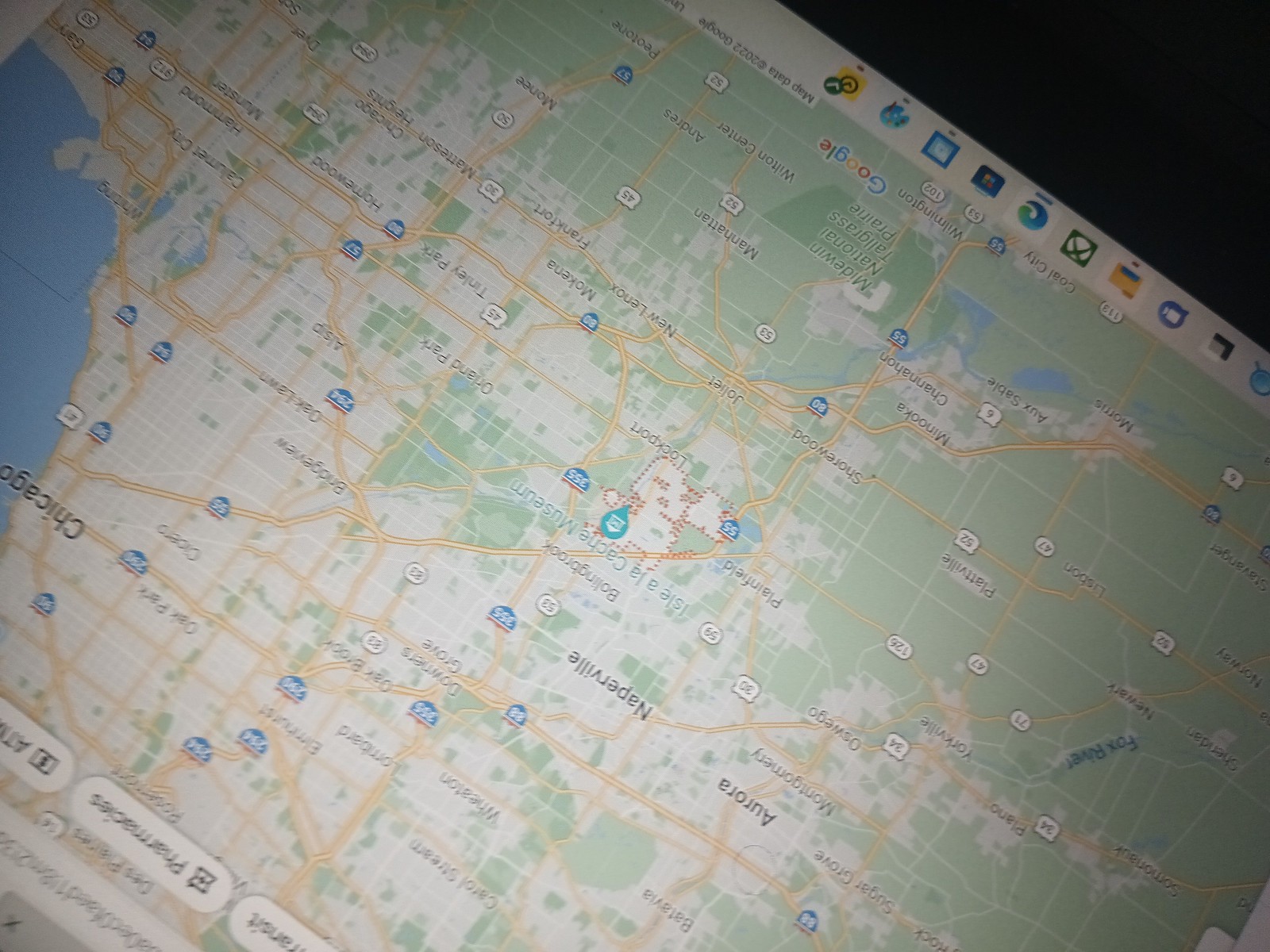The image features an upside-down map set against a dark background. The map itself has a light green backdrop, prominently displaying various geographical and infrastructural details. Towards the left side of the map, there is a depiction of water. The city of Chicago is marked in black letters, with Naperville also labeled. Major interstate highways are represented by thick double red lines, while smaller highways are noted with white signs outlined in black, and their respective numbers are also in black. The land areas on the map are shaded in white or a very light beige and are sometimes outlined in red. Some lakes are colored in green. Additionally, there are small white blocks with black letters spread across the top of the map, and numerous small icons can be found near the bottom.